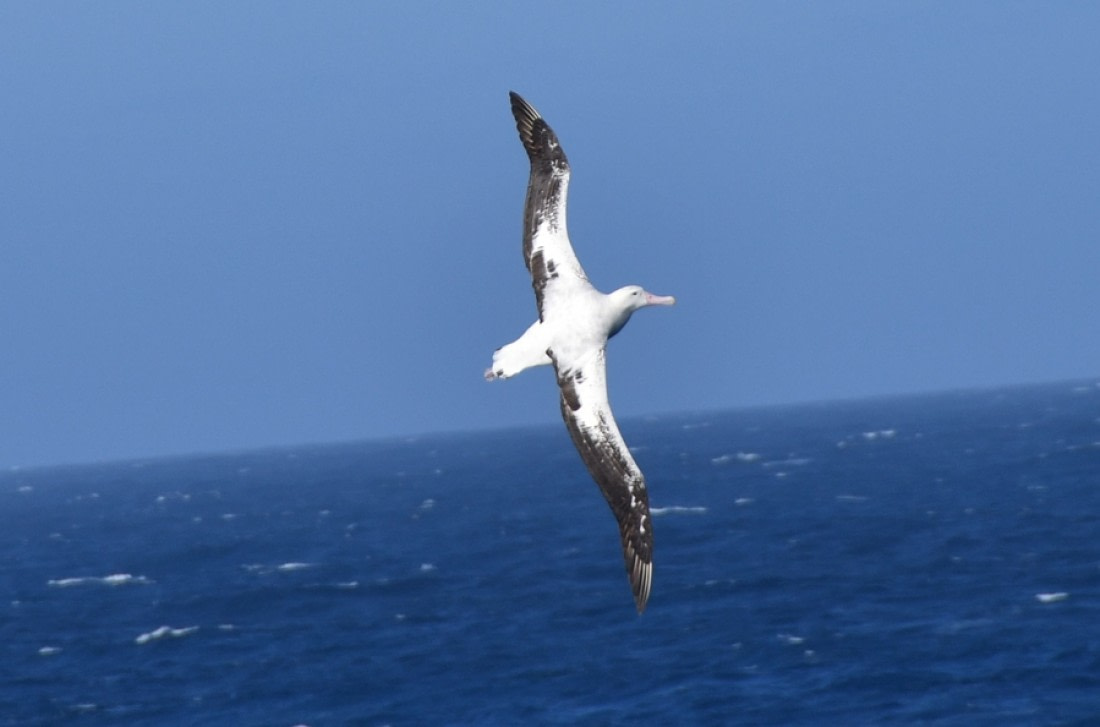A striking image captures a solitary seagull gliding effortlessly over the ocean. The bird, predominantly white with dark gray patterns along the edges of its outstretched wings, features a light pinkish-orange beak and a single black eye. The seagull cuts through a tranquil, cloudless sky that is a vivid blue, mirrored by the slightly darker blue ocean below. Gentle white caps indicate the movement of the ocean's waves. With no other elements in the composition, the scene exudes a sense of peace and simplicity, emphasizing the serene beauty of nature.